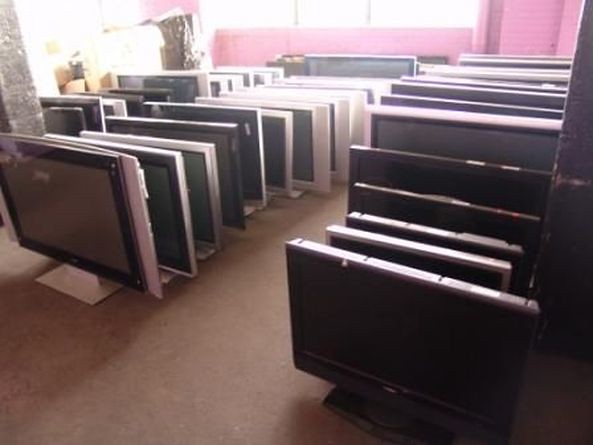This photograph, taken inside a room with a grey floor and pink walls featuring large windows letting in ample light, captures a meticulously arranged display of flat-screen TVs. There are three rows of TVs, each progressively arranged from smaller to larger screens or vice versa. The TVs, approximately 36 to 40 inches in size, are placed on their stands directly on the floor. The TVs vary in appearance, with some in black frames and others in white, giving a sense of variety. While some display what looks like wrappings, this adds to the texture and detail of the scene. The arrangement is neat, with each row of TVs paralleling others, creating a visually compelling and symmetrical composition against the bright, window-lit pink wall.